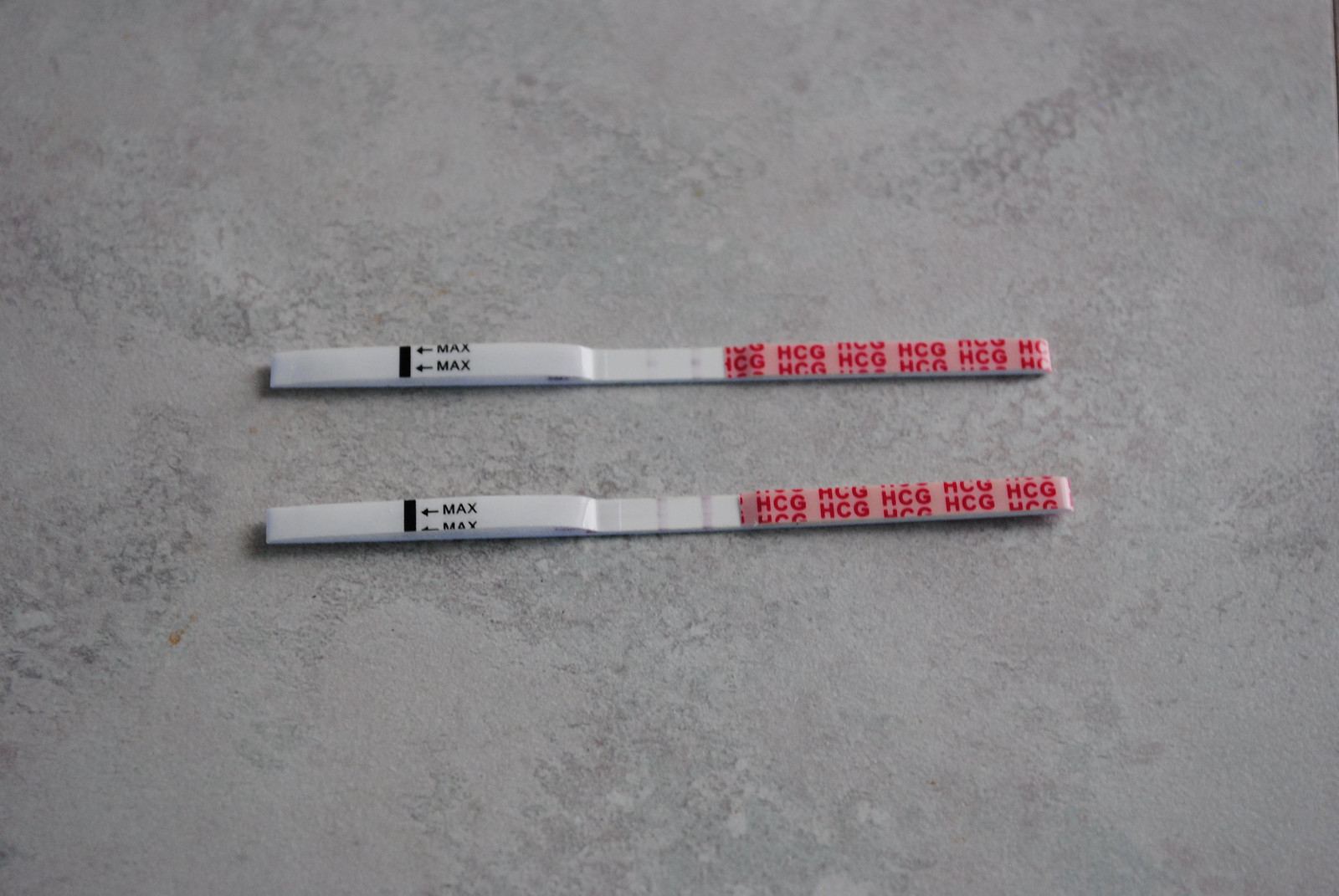The image depicts two adhesive strips, commonly known as command strips, positioned on a grey slab floor. Each strip is equipped with plastic coverings—one featuring the label "HCG" in red text against a pink background, and the other marked with the word "MAX" and two arrows pointing to a black bar. Both coverings are centered and parallel, with about an inch of space between them. Midway on the strips, there is a twist in the adhesive tape.

The grey floor displays a unique texture, seemingly achieved through sponge painting to create a mottled effect. A small brown stain, possibly from a drop of sauce or blood that has oxidized over time, is noticeable on the floor. The scene is evenly illuminated with cool lighting, and there are minimal shadows, providing a clear and detailed view of the elements within the image.